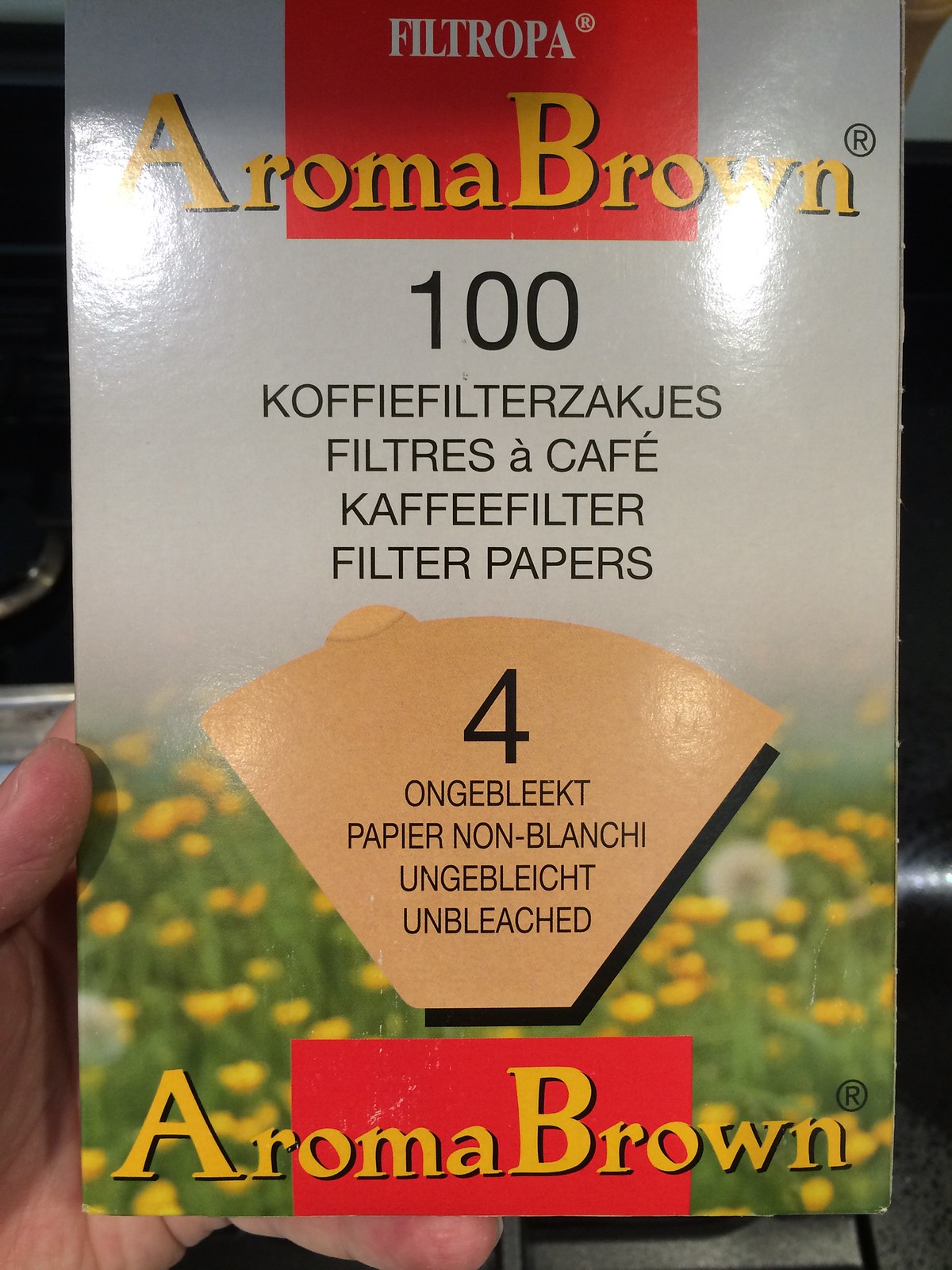This photograph shows a white box of unbleached coffee filter papers. The box prominently displays the brand name "Filtropa" in a red rectangle at the top. Below the brand name, it features a mix of four languages including English, German, Spanish, and another language, detailing the product as unbleached coffee filters. The box also includes the words "Aroma Brown" multiple times, emphasizing the product line. There is a clear image of a coffee filter marked with the number 4, indicating the filter size. A field of yellow daisies decorates the bottom of the box, while a hand is visibly holding up the package in the image.